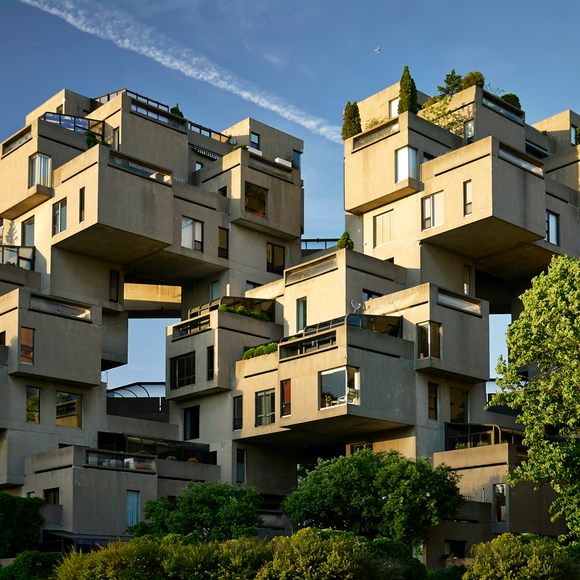This color photograph, taken outside on a clear day with a vivid blue sky, features a uniquely abstract apartment complex. The building, prominent in the image, appears as a staggered, multi-layered structure reminiscent of a Jenga puzzle or a haphazard arrangement of concrete Lego blocks. Its design lacks symmetry, with boxy units jutting out unpredictably in various directions, similar to an intricate ant colony or Tetris pieces assembled without order. The sun illuminates one side of the light brown building, enhancing its three-dimensionality. In the foreground, a hedge line and small trees are visible, while on the right, a taller tree or bush stands. Additionally, there is a vapor trail cutting across the sky, and a distant object, possibly a bird or plane, adds a subtle touch of dynamism to the scene.